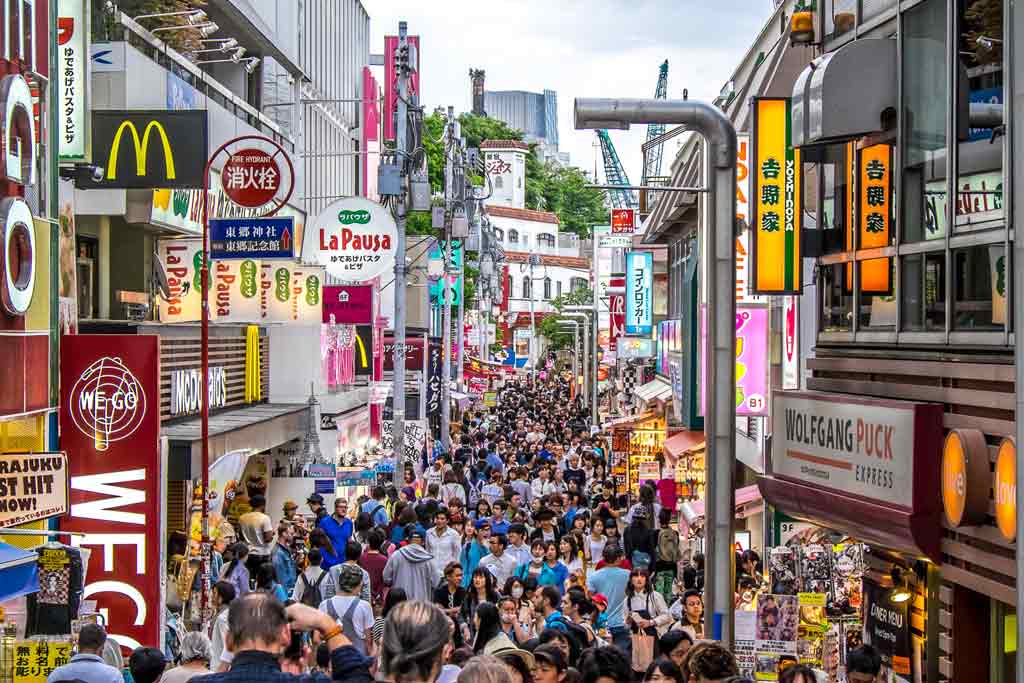This photograph captures the bustling atmosphere of Harajuku in Tokyo, teeming with people packed shoulder-to-shoulder on a lively street. Taken from a slightly elevated perspective, possibly from the second floor of a building, the image showcases shops and restaurants lining both sides of the thoroughfare. Neon signs and Asian letters adorn the storefronts, including familiar names like McDonald's, Yoshinoya, Wolfgang Puck Express, and distinctly Japanese chains such as La Pausa and Wego. In the background, tall buildings and cranes signal ongoing construction in this vibrant area of the city. The diverse crowd, wearing everyday street clothes, navigates the tightly packed street, embodying the dynamic energy of Harajuku.